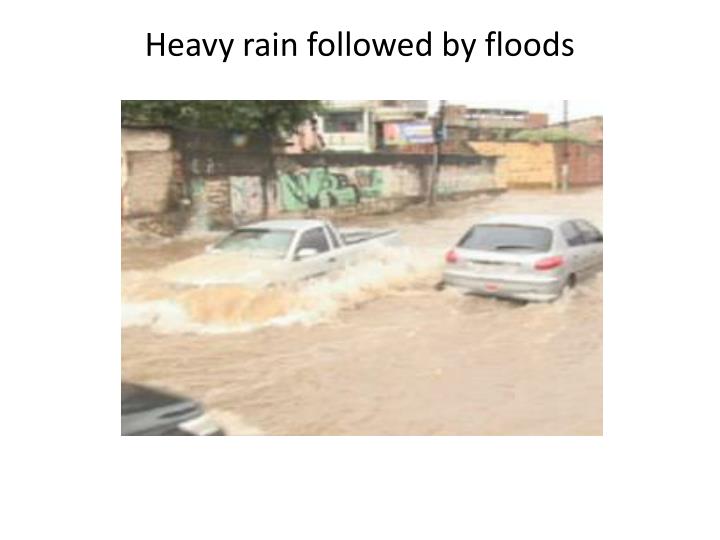The photograph, titled with black text that reads "Heavy rain followed by floods," depicts an urban scene heavily affected by flooding. Three vehicles navigate the flooded streets, with muddy brown water reaching up to the shoulder height of a silver car driving away from the camera, nearly submerging the wheels of a tan pickup truck facing the camera, and partially covering a black vehicle in the lower right corner. In the background, a graffiti-covered wall, adorned with large mint green letters and a black top, indicates a gritty urban environment. Further back, orange and brick red buildings are blurred but suggest a tropical commercial town. The scene is chaotic, capturing the severity of the floodwaters and the struggle of the vehicles pushing through.